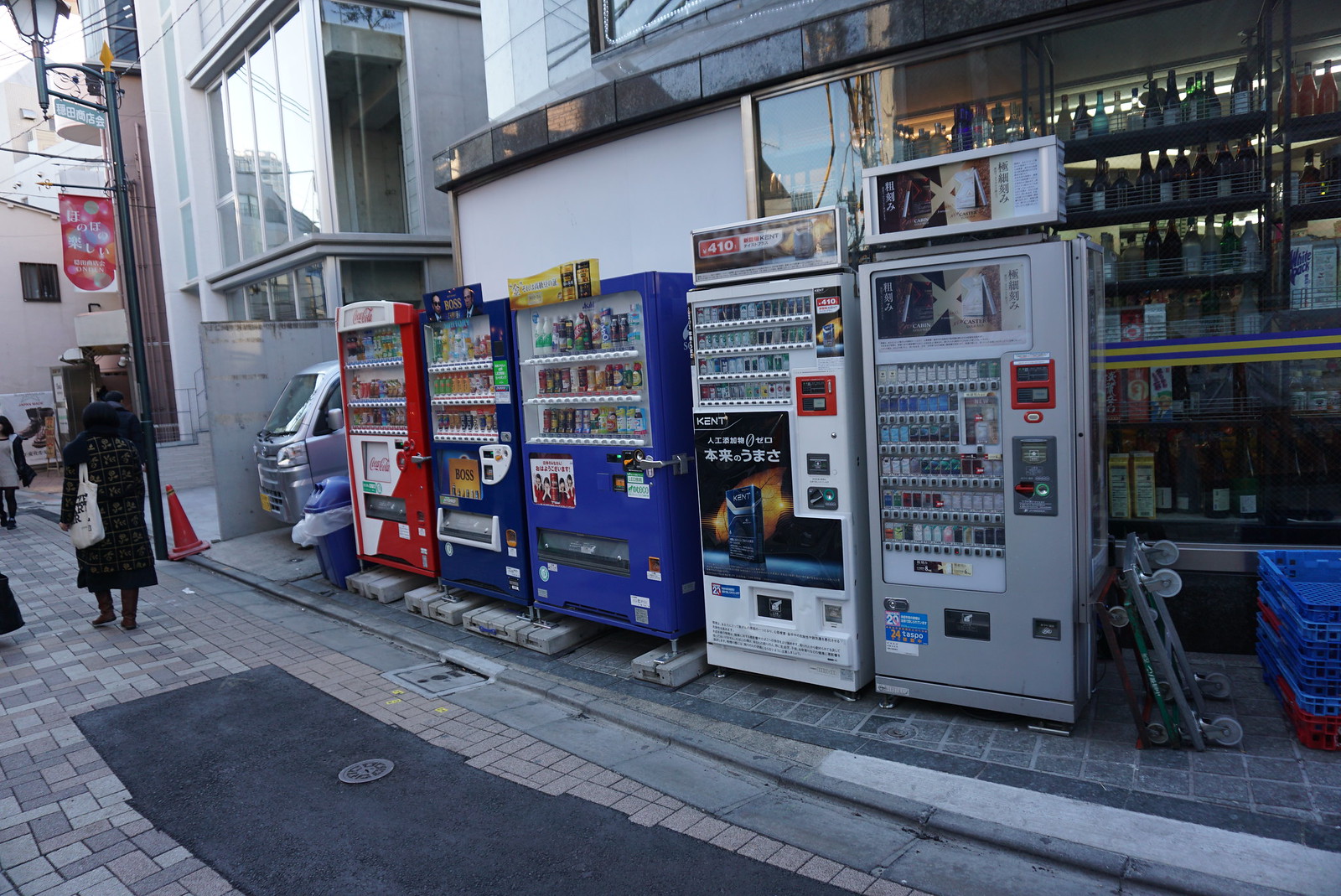The image is a color landscape photograph capturing an urban street scene, presumably in Japan, detailed with mismatched block paving stones in varying shades of dark brown, orange, and sandy white. Among these paving stones are patches of tarmac indicating recent repairs. Alongside a series of mixed-use buildings that serve as both shops and potential residences, a row of five distinct vending machines is lined up on the sidewalk. These vending machines vary in color and style, featuring glass fronts displaying rows of items, likely drinks and bottles. Some vending machines are supported by gray breeze blocks, while others stand tall on their own. Specifics of the vending machines include one red, two blue, a white one with a large poster in Japanese characters, and a grey one with a black-background poster featuring unreadable text in Chinese characters. On the left side of the photograph, a woman in a long black coat with a beige-grey bag over her left shoulder is walking away. Behind the vending machines, part of a grey and blue vehicle is visible. The sidewalk features gray square tiles, adding to the structured yet eclectic aesthetic of the streetscape. Towards the right side, there's a loading area with a grey crate and an upturned object with wheels parked against one of the vending machines. Above and behind the vending machines, windows of an office block can be seen, allowing light to filter through.